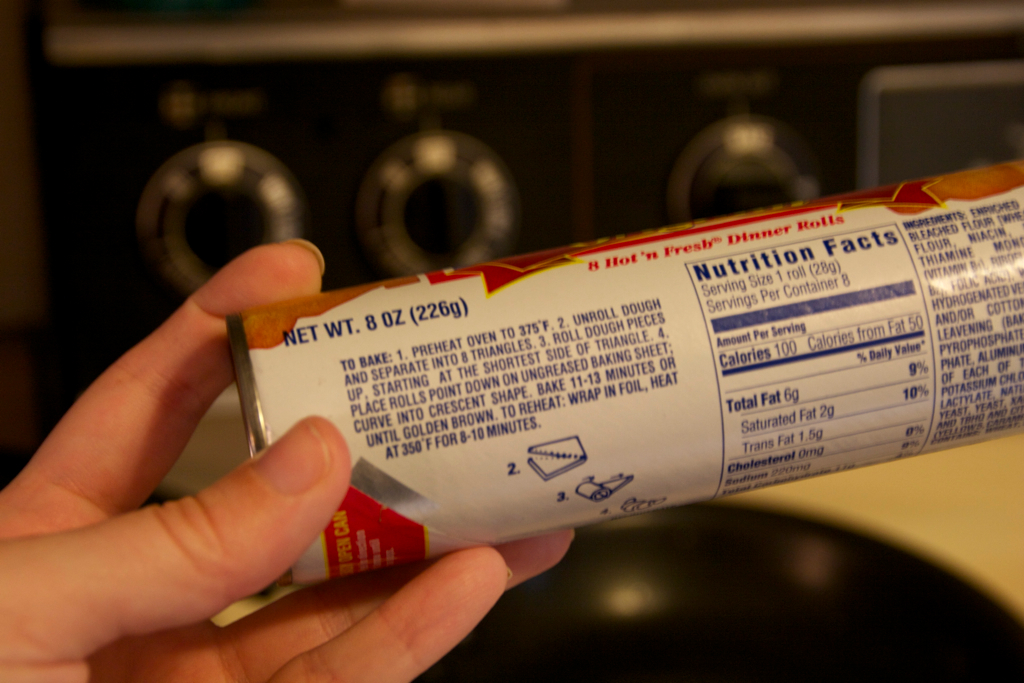This is a color photograph of a can of dinner rolls being held by a Caucasian hand in front of an older-style stove range. The can, which features a design in white, brown, and red, prominently displays the text "8 Hot and Fresh Dinner Rolls" and specifies a net weight of 8 ounces (226 grams). The blue text on the white background also indicates nutritional facts, with a serving size of one roll and eight servings per container, each containing 100 calories. To the right side of the can, the detailed cooking instructions read: "Preheat oven to 375°F. Unroll dough and separate into triangles. Roll dough pieces up, starting at the shortest side of the triangle. Place rolls point down on an ungreased baking sheet, curve into a crescent shape. Bake for 11 to 13 minutes or until golden brown." The image captures the can’s intricate details and the hand holding it, with the blurred background revealing an oven and a black pan, adding a domestic kitchen ambiance.